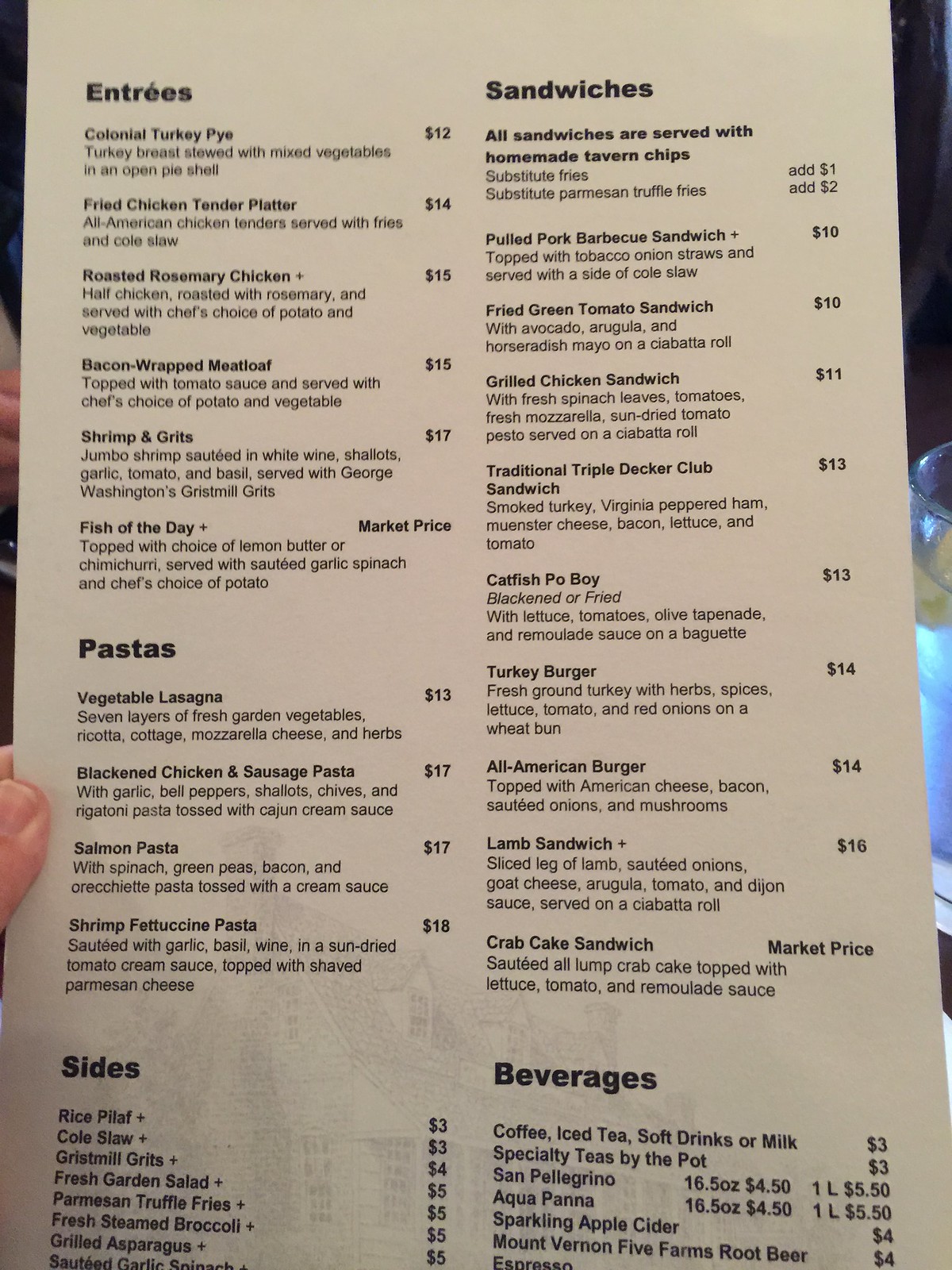The image showcases a neatly arranged menu held by someone, divided into two distinct columns with five main headers: Entrees, Sandwiches, Pastas, Sides, and Beverages. The left column begins with the Entrees section, listing six delectable options: Colonial Turkey Pie, Fried Chicken Tender Plate, Roasted Rosemary Chicken, Bacon-Wrapped Meatloaf, Shrimp and Grits, and Fish of the Day, each accompanied by prices and detailed descriptions. 

Following the entrees is the Pastas section, featuring Vegetable Lasagna, Blackened Chicken and Sausage Pasta, Salmon Pasta, and Shrimp Fettuccine Pasta, all described and priced accordingly. Below the pastas, the Sides section offers an array of choices including Rice Pilaf, Coleslaw, Gristmas Grits, Fresh Garden Salad, Parmesan Truffle Fries, Grilled Asparagus, and Sautéed Garlic.

In the right column, the Sandwiches section indicates that all sandwiches come with homemade tavern chips, with an option to substitute for Parmesan Truffle Fries. The sandwiches, each with detailed descriptions and prices, include Pulled Pork Barbecue Sandwich, Fried Green Tomato Sandwich, Grilled Chicken Sandwich, Traditional Triple Deck Club Sandwich, Catfish Po' boy, Turkey Burger, All American Burger, Lamb Sandwich, and Crab Cake Sandwich.

Finally, the Beverages section lists Coffee, Tea, Soft Drinks or Milk, Specialty Teas, Water Options, Root Beer, and Espresso.